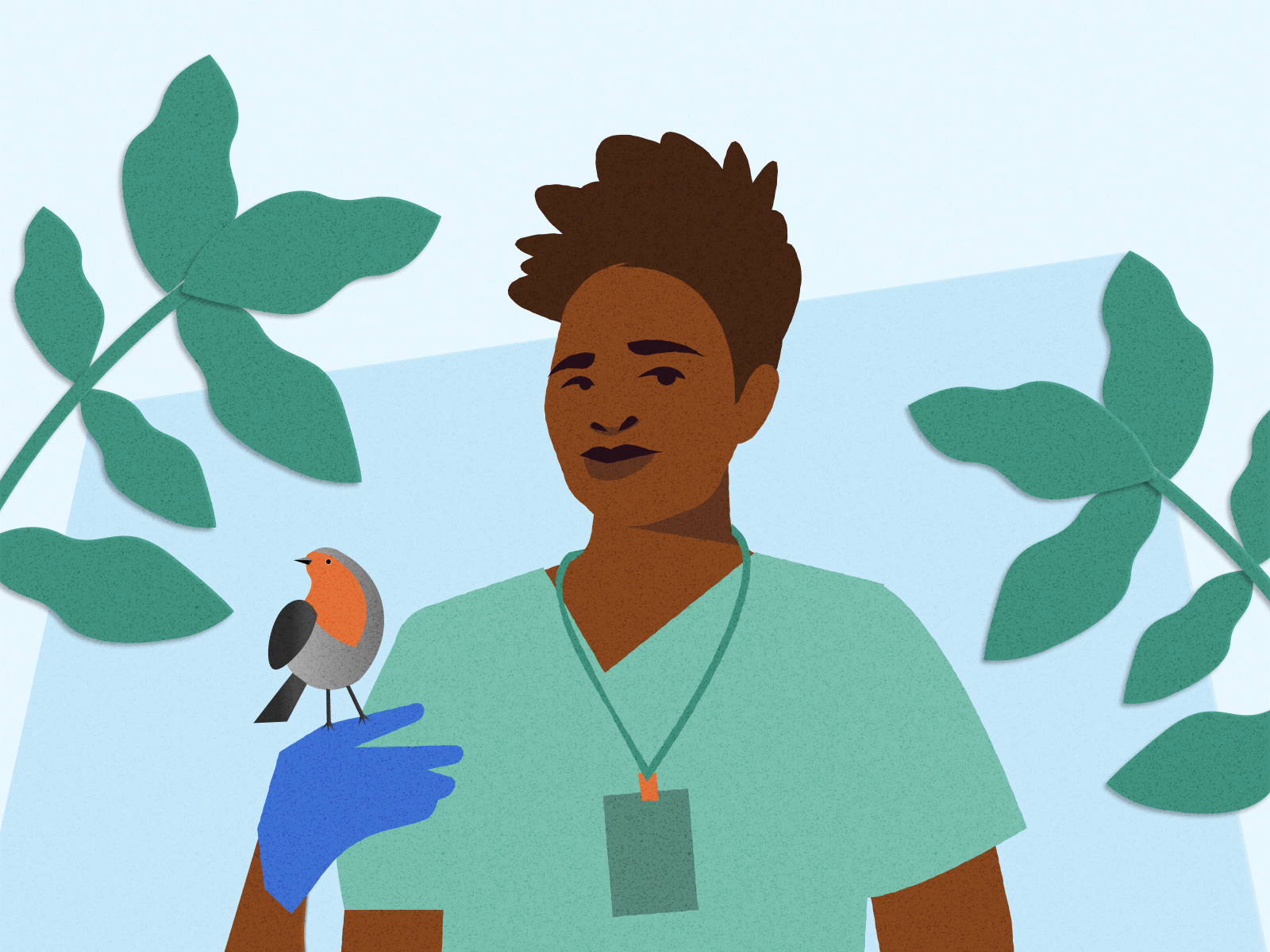The image is a modern digital drawing, characterized by a simple, almost cut-out paper aesthetic. It centers on a dark-skinned man, possibly a nurse, wearing green scrubs and a lanyard with an orange clip. He has short, spiky dark hair and appears to be smirking slightly while looking at the viewer. His left hand, adorned with a blue latex glove, is raised with a perched bird on his finger. The bird features black wings and a tail, a gray stomach and neck, and an orange face. The background is light blue with houseplants and large leaves flanking the man on both sides, adding a touch of greenery to the predominantly white, blue, and green scene.